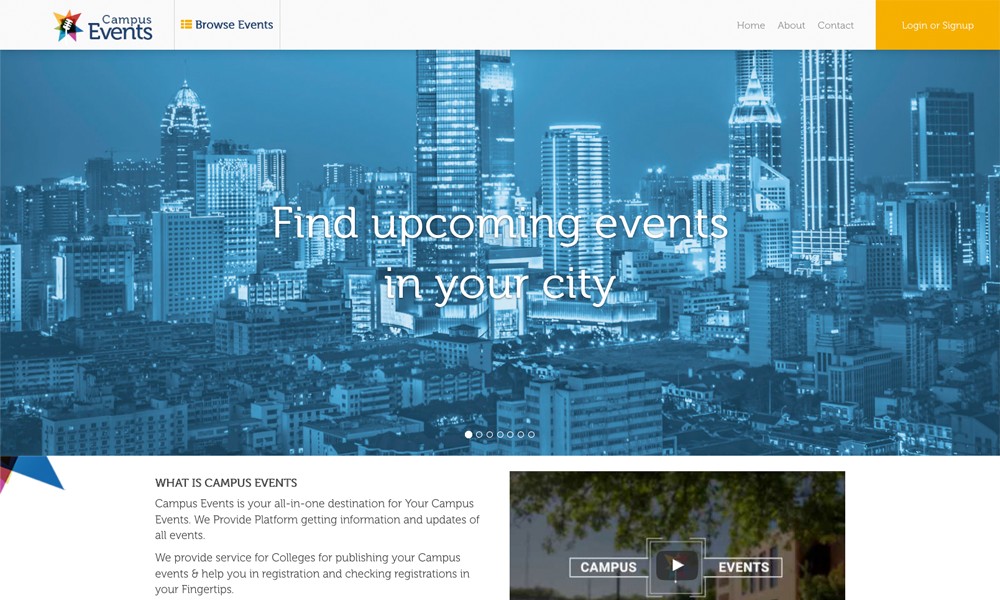Sure, here's a detailed and cleaned-up caption for the provided image description:

---

This image depicts the front page of a website dedicated to campus events. In the upper left corner, the website prominently displays its name, "Campus Events," along with its vibrant logo, which resembles a firework bursting in yellow, red, blue, and purple hues, centered by a white tack. Adjacent to the logo, the phrase "Browse Events" is clearly visible. 

On the right-hand side of the navigation bar, you'll find links labeled "Home," "About," "Contact," followed by options to "Log In" or "Sign Up."

Below the navigation bar, a captivating photograph of a city skyline at nighttime, overlaid with a subtle blue tint, serves as the page's header. Emblazoned across the photo is the invitation, "Find upcoming events in your city." 

Further down, a section titled "What is Campus Events?" provides a succinct introduction to the platform. It explains that Campus Events is a comprehensive tool designed to keep users informed about campus happenings. The platform not only helps colleges publish event details but also offers services to facilitate event registration and management, all accessible at your fingertips.

To the right of this informative text, there's a clickable video thumbnail featuring an outdoor snapshot labelled "Campus Events." This video offers an overview of the platform's capabilities, demonstrating how it assists colleges in listing events and enables students to discover various happenings in their city and on their campus.

---